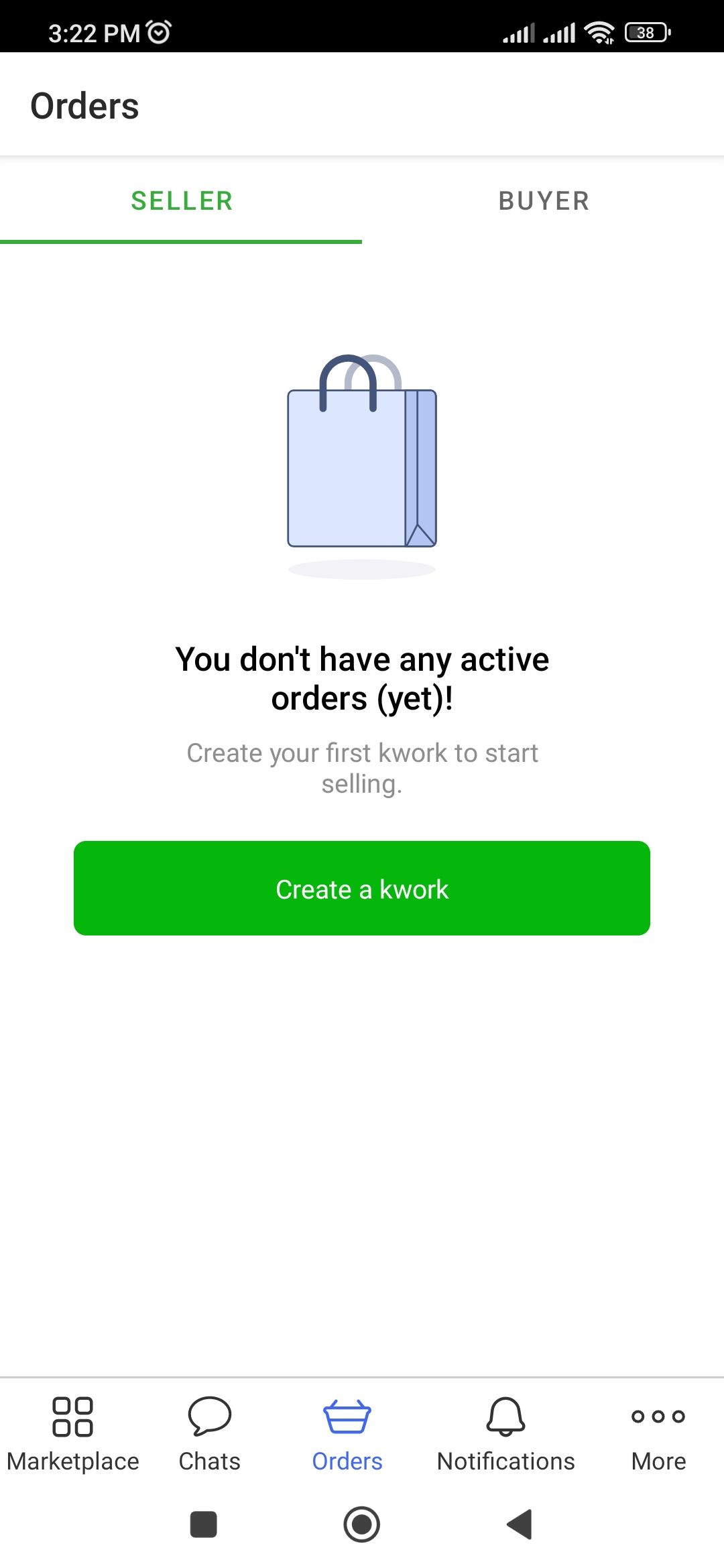In this detailed image, you can see the screen of an Android device. At the very bottom of the screen are several navigation icons typical of such devices. Starting from the left, the first icon is the "Recent Apps" icon, followed by a circular "Home" button at the center, and a left-facing triangle functioning as the "Back" button.

Along the top edge of the screen is a black bar displaying white text and icons. On the left side of this bar is the current time, "3:22 PM", accompanied by an alarm clock icon. On the right side, there are two service bars, a Wi-Fi signal icon, and a battery icon displaying a 38% charge.

Below this black bar is a title in black text that reads "Orders" against a white background. A thin gray horizontal line separates this title from the rest of the screen. Directly below this line are two buttons; the first button is green and labeled "Seller" with a green border underneath the text, and the second button is labeled "Buyer" in black text with no border.

In the central part of the page is an illustration of a light blue and dark blue shopping bag. Beneath this illustration, black text reads: "You don't have any active orders (yet). Create your first K-Work to start selling." This message encourages the user to take action. Further down, there is a large green rectangular button with white text that reads "Create a K-Work".

At the very bottom of the screen are more icons in gray, each labeled accordingly. From left to right, these icons are: "Marketplace" (represented by a grid of squares), "Chats" (speech bubble), "Orders" (shopping basket), "Notifications" (bell), and "More" (ellipses, represented by three dots).